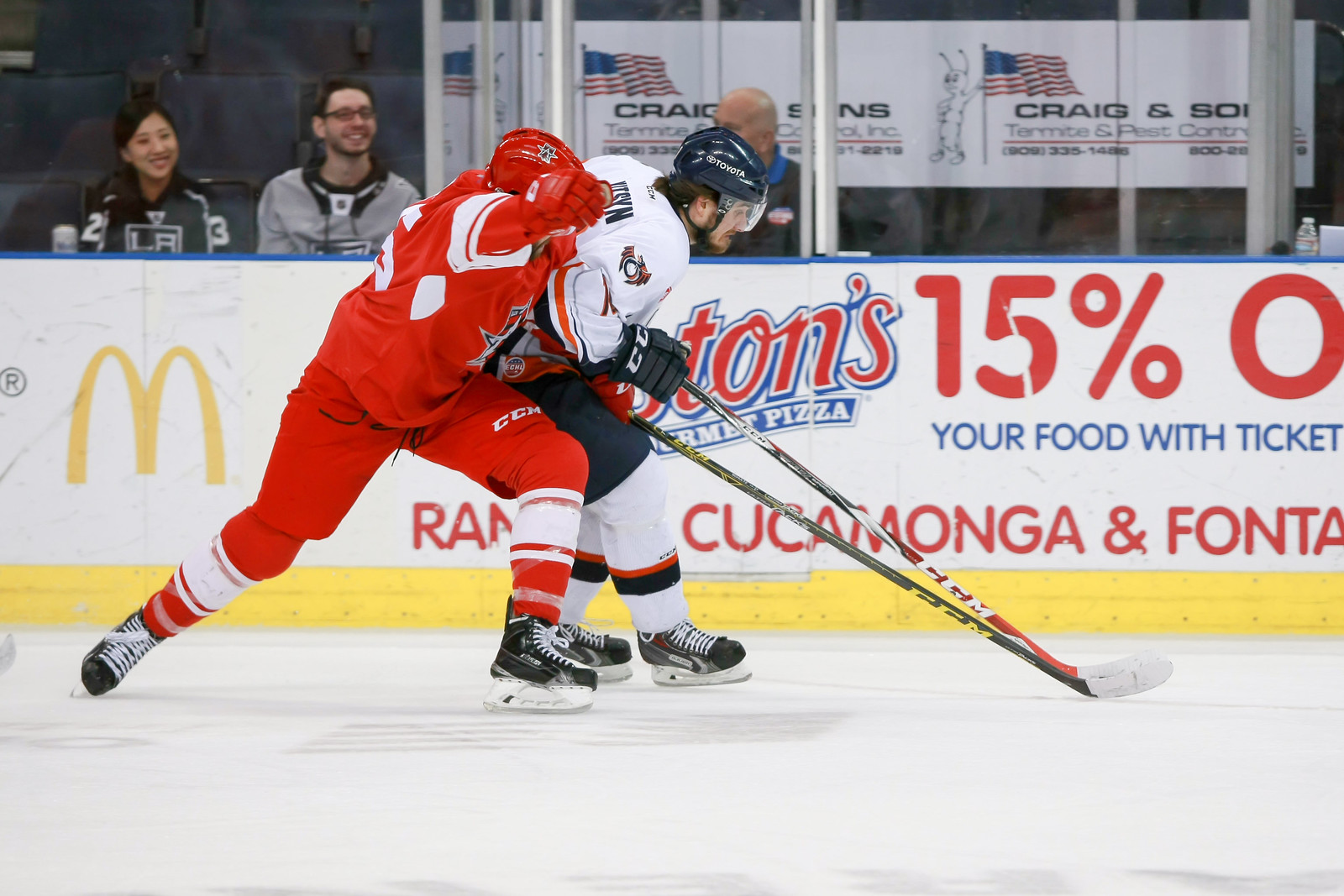In this close-up image of a heated ice hockey game, two players are battling for control of the puck. The player on the left, dressed in a deep red uniform with black skates, contrasts with his opponent to the right, who sports a white jersey and blue helmet, complemented by blue shorts over heavy protective pants. Their hockey sticks are locked in a tense struggle, tips touching as they both reach for the puck on the ice. The scene is set against a short barrier wall adorned with advertisements, prominently featuring brands like McDonald's and Craig and Sons, with some displaying patriotic American flags, suggesting a game likely held in California, indicated by city names such as Fontana. Above the barrier, a protective plastic shield separates the rink from the spectators. Among the crowd, a man and a woman are visibly engaged, smiling and enjoying the game, adding a lively atmosphere to the intense on-ice action.